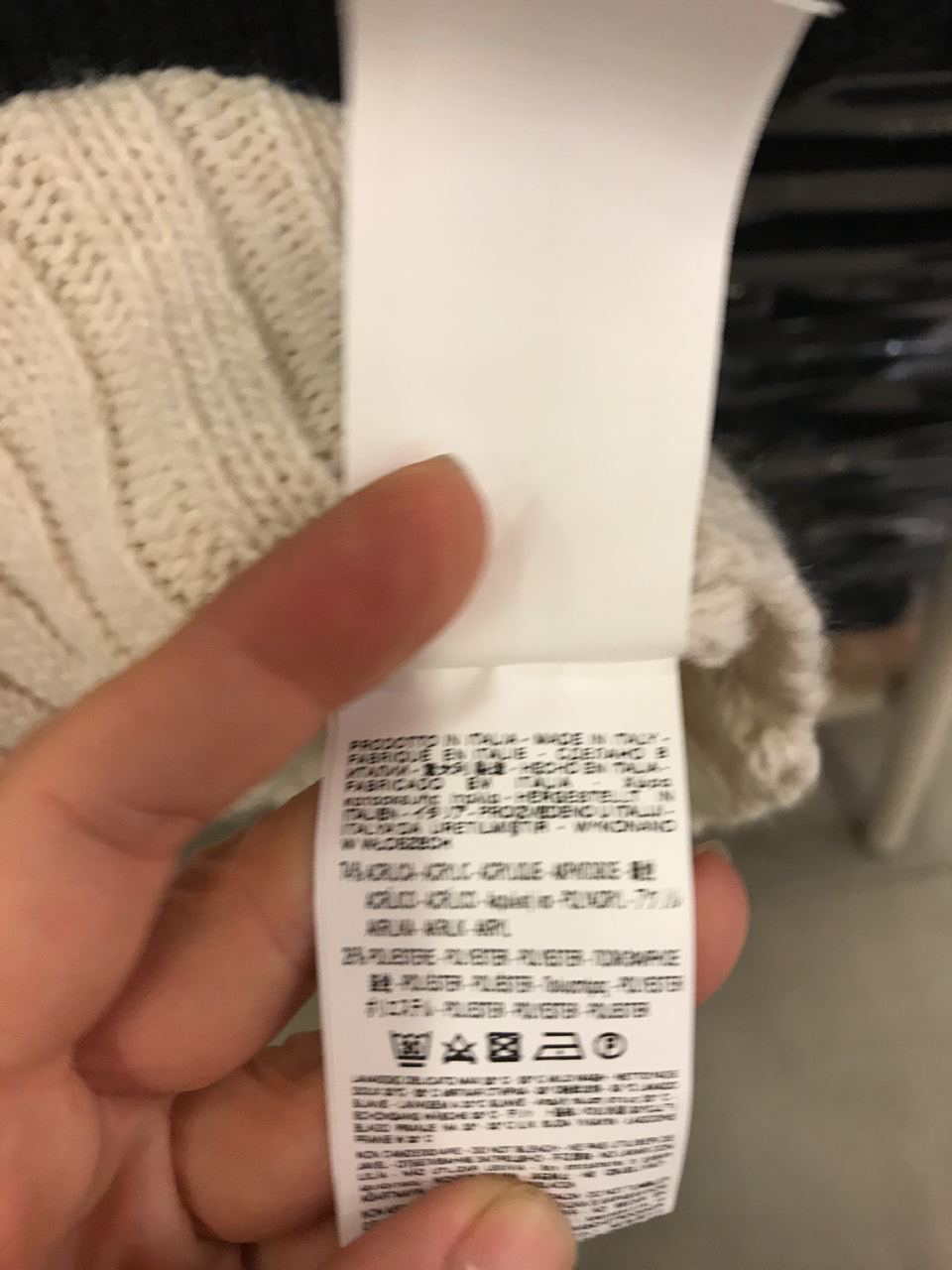This image depicts a close-up photograph of a laundry tag attached to a cream-colored knitted item, which could be a beanie or a sweater. The tag, white with black text that is unreadable due to the image being out of focus, provides care instructions for the garment. The knitted item features a textured pattern of alternating rows of knits and purls, arranged in a grid-like three-by-three formation. In the foreground, a hand with its palm upward holds the tag; the thumb and pinky securing it while one finger rests over the crease. The background reveals light-colored flooring along with some indistinct elements that may include black shelving on one side and possibly the legs of a chair and a table on the other.